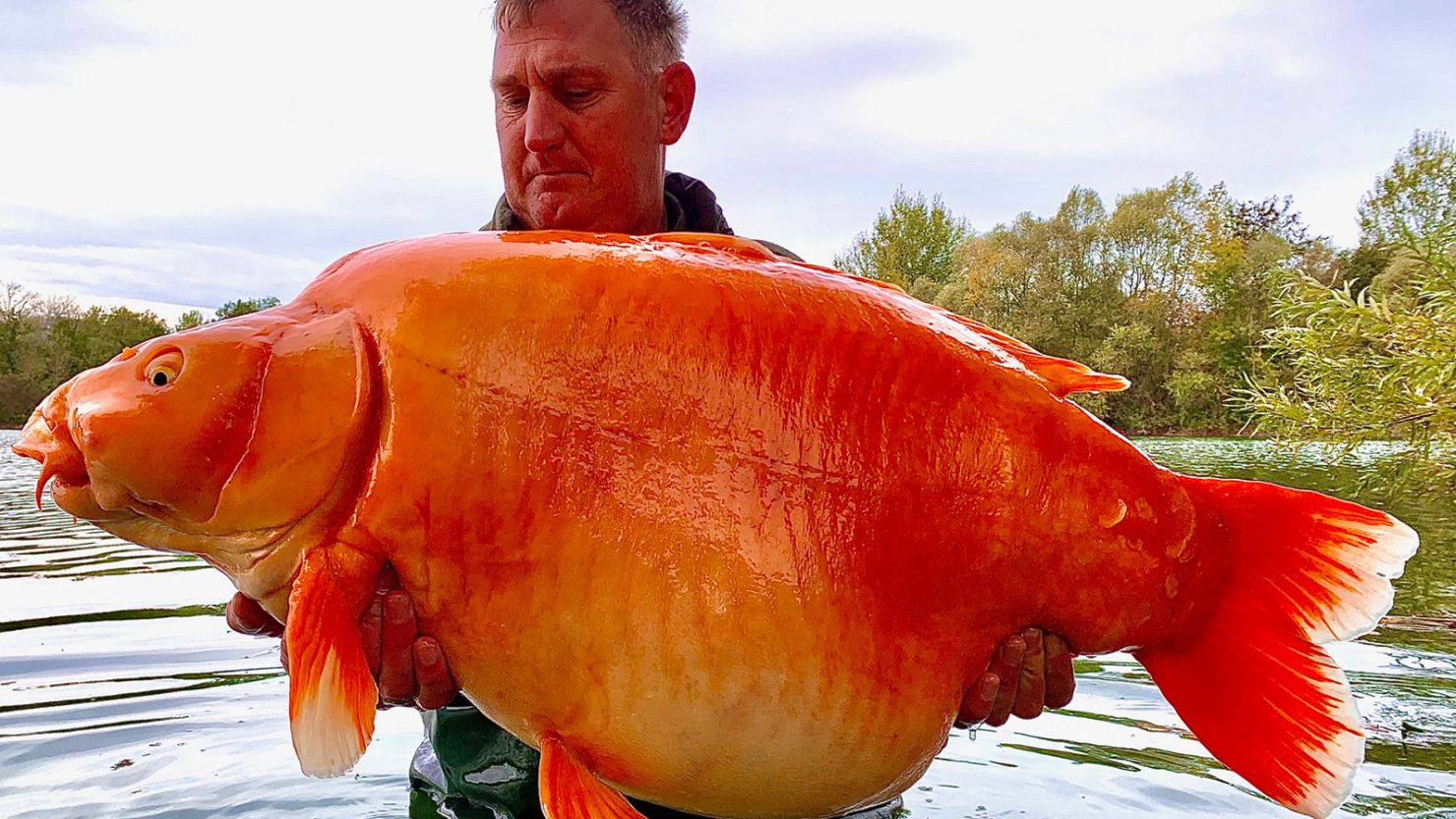In this image, a Caucasian male is prominently displayed holding a large goldfish. The fish is quite substantial in size, notably bright orange in color with a particularly swollen belly that hangs noticeably. The man is gripping the fish firmly, with one hand positioned under the front fins and the other supporting it from behind the belly. He stands in front of a vast body of water, presumably where he caught the fish, with gentle waves and a flowing current visible in the background. Surrounding the body of water are lush trees adorned with vibrant green leaves. The man gazes down at the fish, seemingly inspecting his impressive catch.